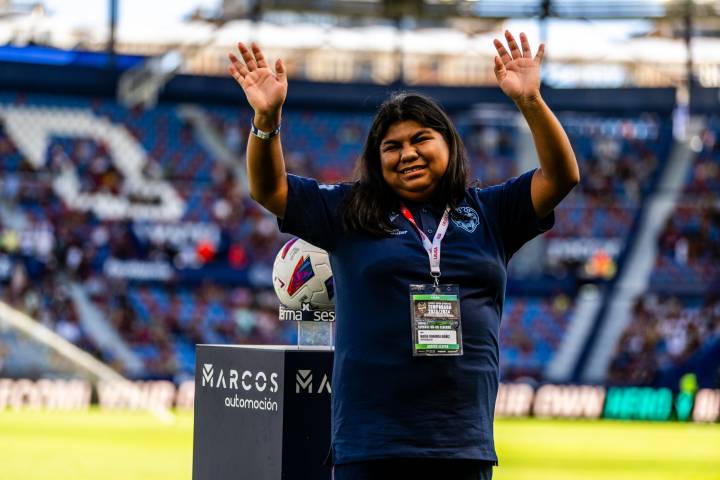In this rectangular image taken at a sports stadium, the predominant colors are various shades of blue and white, with elements of green from the turf. At the center of attention is a woman of likely Mexican or Guatemalan descent who appears to be in her late 40s and slightly overweight. She has shoulder-length dark hair and is seen smiling with her hands raised above her head, palms outstretched, giving the impression she is celebrating a victory. She is dressed in a dark blue short-sleeved shirt and black trousers. Around her neck, she wears a lanyard with a large plastic badge, possibly indicating credentials or special access.

To her right, on a square black pedestal that bears the partial text "Marcos Otto Messiaen," rests a soccer ball in a trophy-type configuration. This pedestal stands out prominently. The background features stadium stands that are partially filled with fans, creating a blurred effect. Some stadium seats appear blue and red, though the stands are not crowded. At the lower part of the image, the light green field is visible, along with some blurred advertisements on the surrounding wall. At the very top of the image, a fenced-off walkway can be seen, adding to the stadium atmosphere.